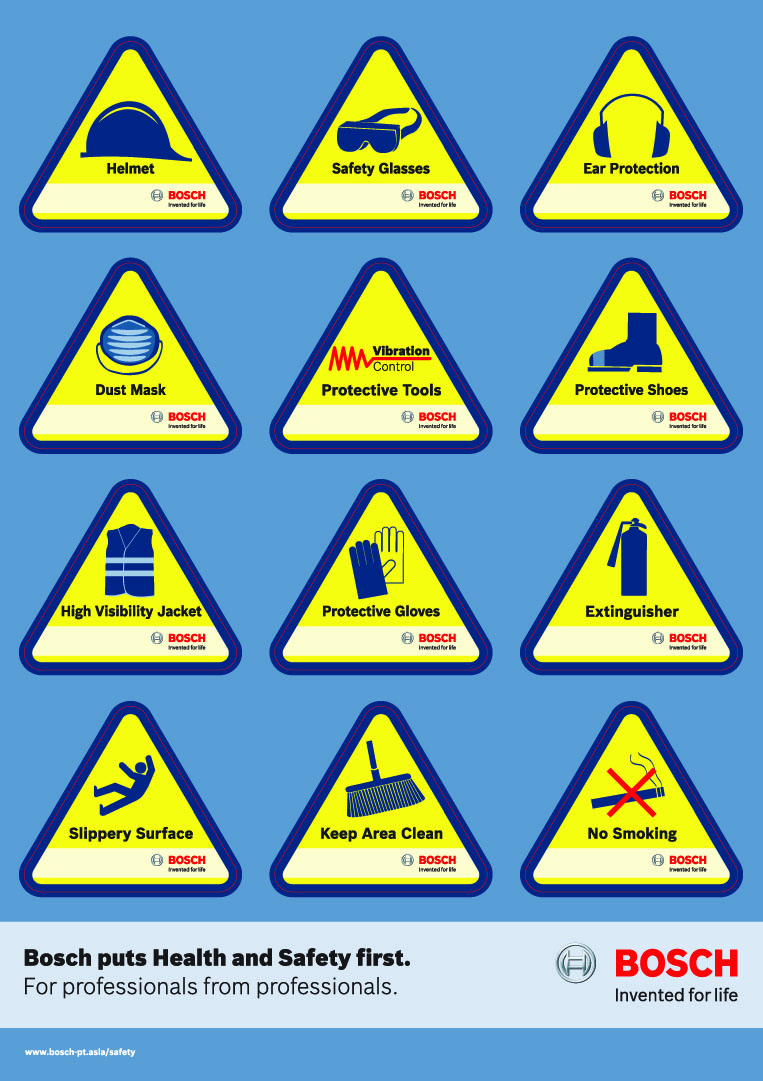This vertically aligned rectangular image features a comprehensive safety signage flyer against a solid blue background. It is divided into four rows with three triangular signs in each row, all outlined in dark blue, with a yellow upper and middle section and a white section at the bottom. Each triangle contains relevant Bosch safety guidelines and illustrations.

Starting from the top left, the signs depict:
1. A blue helmet labeled "Helmet."
2. Blue safety glasses labeled "Safety Glasses."
3. Blue ear protection labeled "Ear Protection."

The second row features:
4. A dust mask labeled "Dust Mask."
5. A zigzag line with the words "Vibration Control."
6. A protective boot labeled "Protective Shoes."

The third row displays:
7. A high visibility jacket with the label "High Visibility Jacket."
8. Protective gloves showing a blue and a white glove labeled "Protective Gloves."
9. An extinguisher labeled "Extinguisher."

The final row includes:
10. A person slipping labeled "Slippery Surface."
11. A broom labeled "Keep Area Clean."
12. A red X over a cigarette labeled "No Smoking."

At the bottom, the flyer states, "Bosch puts health and safety first for professionals from professionals," with "BOSCH" in red capital letters. Below that, it reads, "Invented for life."